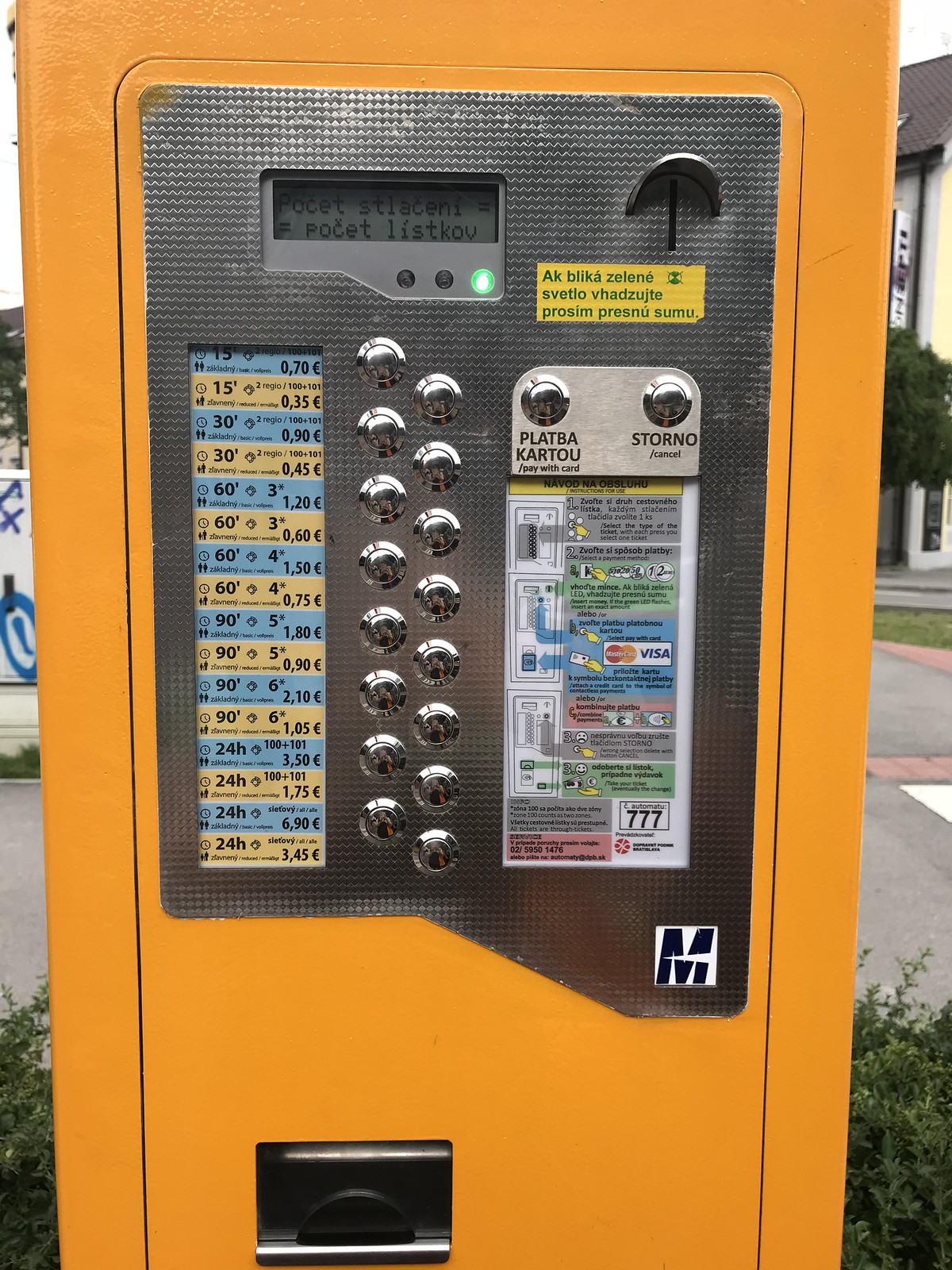The image depicts an orange metal kiosk designed for purchasing parking tickets. The device, which stands relatively tall, features a prominent silver panel covering a significant portion of its front. At the top, a hooded coin slot can be seen, along with a coin slot sign in an unidentified Eastern European language, possibly Polish or Czech. Below the coin slot, there’s an LCD screen displaying unreadable text, and a reassuring green button indicating operational status. The machine also includes an array of silver buttons on the left, which resemble elevator buttons, correlating with the tiered pricing structure displayed next to them. Prices, listed in euros, suggest options for different parking durations ranging from hourly rates to full-day rates. Noteworthy details include a Visa and MasterCard logo for card transactions, an instructional card showing how to insert payment cards, and a physical slot at the bottom likely for dispensing tickets, change, or receipts. The device, which might also be used for purchasing metro tickets, includes a number to call for assistance and a decal with a letter 'M' on the bottom right of the silver panel.